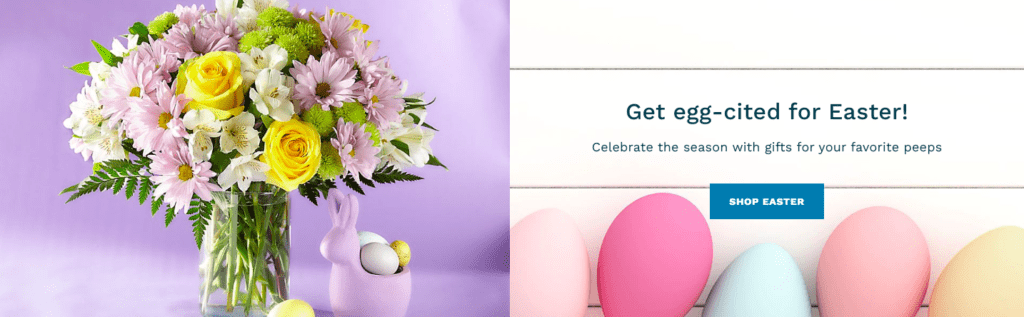A vibrant Easter-themed advertisement decorates the webpage, divided into two visually appealing sections. On the left, a stunning flower arrangement captures attention with its varied hues. Dominated by blooms in shades of purple, white, and pink, the arrangement also features two striking yellow roses and lush greenery, all elegantly displayed in a clear vase. Beside this colorful bouquet, a charming ceramic dish shaped like a bunny sits proudly. The bunny dish, complete with a cute head and distinctive ears, holds three festive Easter eggs in its back: one white, one purple, and one yellow.

On the right side of the webpage, cheerful text invites visitors to "Get Egg-cited for Easter." The message encourages people to "Celebrate the season with gifts for your favorite peeps," and directs them to "Shop Easter" through a convenient search bar. Below the cheerful text, a row of five brightly colored eggs echoes the holiday spirit. The eggs come in a palette of white, dark purple, light blue, pink, and yellow, enhancing the overall festive atmosphere of this enticing Easter advertisement.